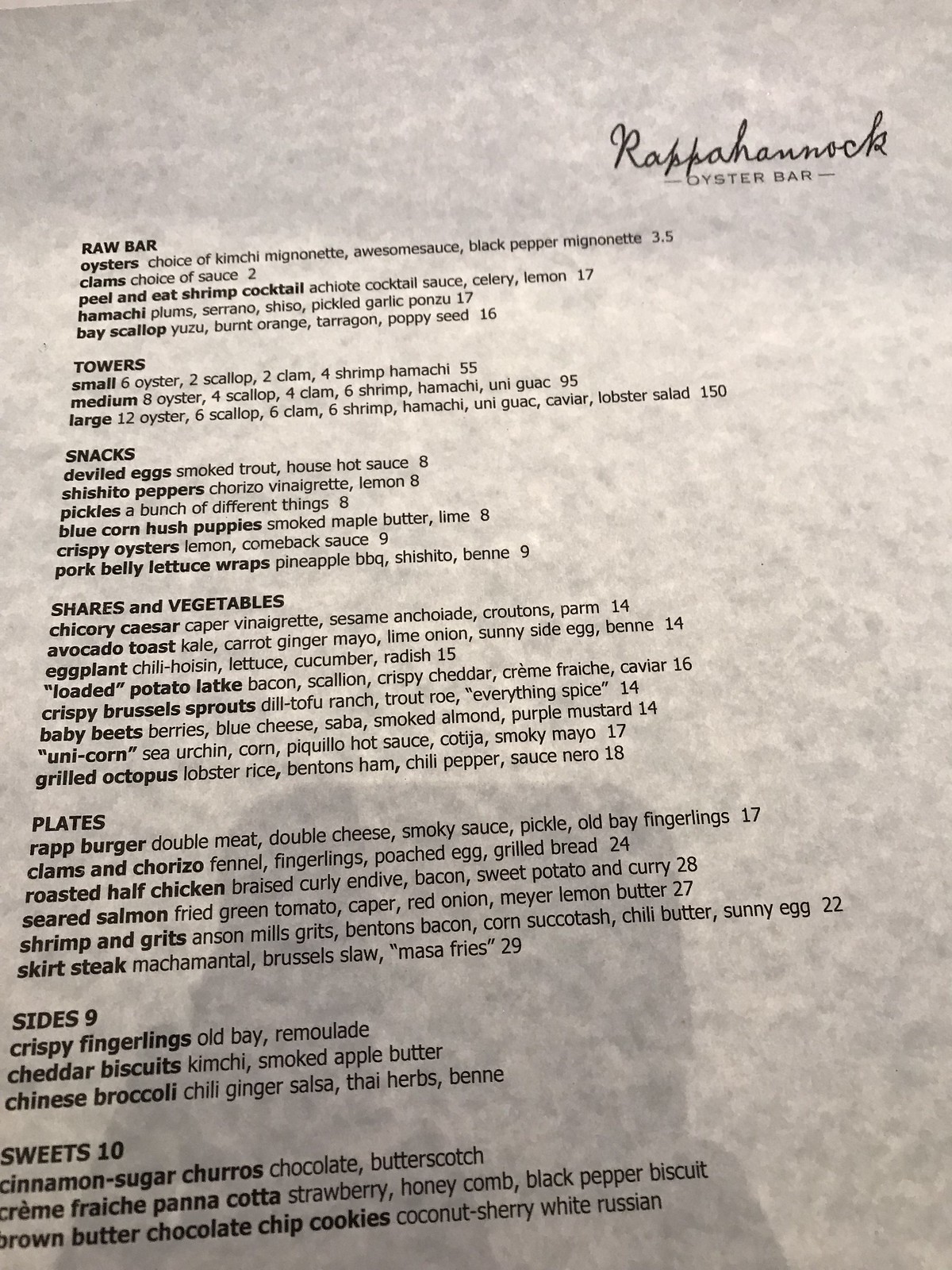The menu from Rappahannock Oyster Bar is printed on grey, textured paper and photographed at an angle, making the nearer entries appear larger than the farther ones. The text is in black Tahoma font, with menu items bolded, headings in block capitals, and individual items in lowercase. The sections are: RAW BAR, TOWERS, SNACKS, SHARES AND VEGETABLES, PLATES, SIDES 9, and SWEETS 10.

**RAW BAR:**
- Oysters: choice of kimchi, mignonette, awesome sauce, black pepper mignonette, $3.50 each
- Clams: choice of sauce, $2 each
- Peel-and-eat shrimp cocktail: achiote cocktail sauce, celery, lemon, $17
- Hamachi: plums, serrano, shiso, pickled garlic ponzu, $17
- Bay scallop: yuzu, burnt orange, tarragon, poppy seed, $16  

**TOWERS:**
- Small: 6 oysters, 2 scallops, 2 clams, 4 shrimp, hamachi, $55
- Medium: 8 oysters, 4 scallops, 4 clams, 6 shrimp, hamachi, uni guac, $95
- Large: 12 oysters, 6 scallops, 6 clams, 6 shrimp, hamachi, uni guac, caviar, lobster salad, $150  

**SNACKS:**
- Deviled eggs: smoked trout, house hot sauce, $8
- Shishito peppers: chorizo vinaigrette, lemon, $8
- Pickles: assorted, $8
- Blue corn hushpuppies: smoked maple butter, lime, $8
- Crispy oysters: lemon, comeback sauce, $9
- Pork belly lettuce wraps: pineapple barbecue, shishito, benne, $9  

**SHARES AND VEGETABLES:**
- Chicory Caesar: caper vinaigrette, sesame enchilada, croutons, parm, $14
- Avocado toast: kale, carrot ginger mayo, lime, onion, sunny-side egg, benne, $14
- Eggplant: chili hoisin, lettuce, cucumber, radish, $15
- Loaded potato latkes: bacon, scallion, crispy cheddar, crème fraîche, caviar, $16
- Crispy Brussel sprouts: dill tofu ranch, trout roe, “everything spice,” $14
- Baby beets: berries, blue cheese, saba, smoked almond, purple mustard, $14
- “Unicorn” sea urchin: corn, pequillo, hot sauce, cotija, smoky mayo, $17
- Grilled octopus: lobster, rice, Betterton's ham, chili pepper, salsinero, $18  

**PLATES:**
- Wrapped burger: double meat, double cheese, smoky sauce, pickle, Old Bay fingerlings, $17
- Clams and chorizo: fennel, fingerlings, poached egg, grilled bread, $24
- Roasted half chicken: braised curly endive, bacon, sweet potato and curry, $28
- Seared salmon: fried green tomato, capers, red onion, mayo, lemon butter, $27
- Shrimp and grits: Anson Mill grits, Fenton's bacon, corn succotash, chili butter, sunny-side egg, $22
- Skirt steak: mashed mantel, brussels slaw, “masa fries,” $29  

**SIDES (each $9):**
- Crispy fingerlings: Old Bay and remoulade
- Cheddar biscuits: kimchi, smoked apple butter
- Chinese broccoli: chili ginger salsa, Thai herbs, benne  

**SWEETS (each $10):**
- Cinnamon sugar churros: chocolate butterscotch
- Crème fraîche panna cotta: strawberry honeycomb
- Black pepper biscuit: brown butter chocolate chip cookies
- Coconut sherry: white Russian  

The image also features a shadowed area at the bottom of the menu, with lighting highlighting up to the top of the RAW BAR section, gradually dimming towards the logo in the upper right-hand corner.